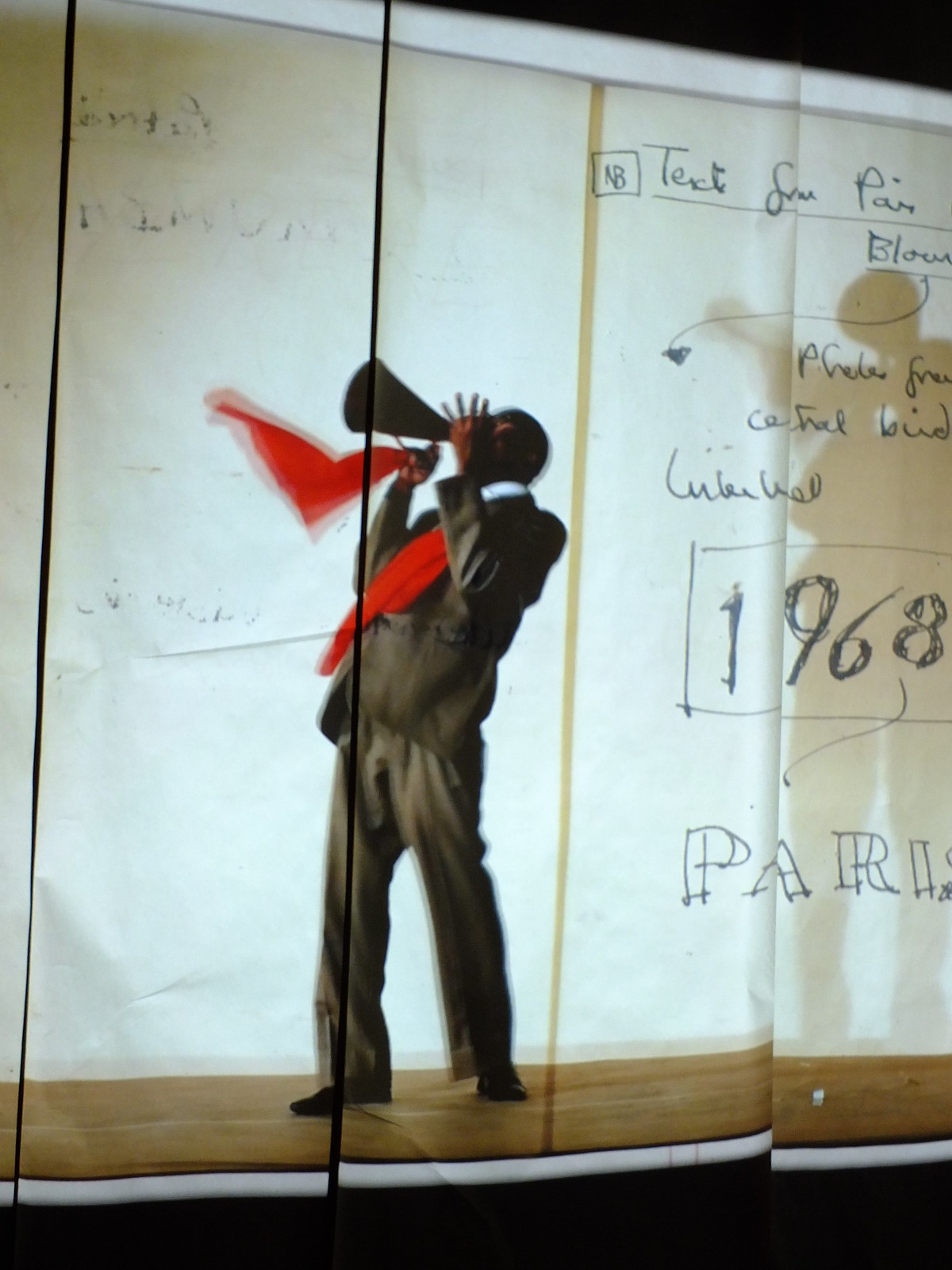This color photograph depicts a mural artwork displayed in portrait orientation, spanning three vertical panels. The illustration features a man standing on a wooden floor, turned to the left, partially obscuring his face with his raised left hand. He is attired in a brown suit, white shirt, and a red tie or scarf. In his right hand, he holds a black megaphone, which stands out against the otherwise subdued colors. The background of the image comprises a white canvas-like surface, divided into sections with visible vertical lines. On the right side of the artwork, there is scribbly handwriting with large numbers '1968' prominently displayed. The visual style combines elements of photographic realism with a blurry, slightly unfocused quality, giving it a motion-like effect. Shadows cast along the top and bottom edges contribute to the dramatic composition, while the handwritten notes hint at historical or cultural references, possibly relating to Paris in 1968.